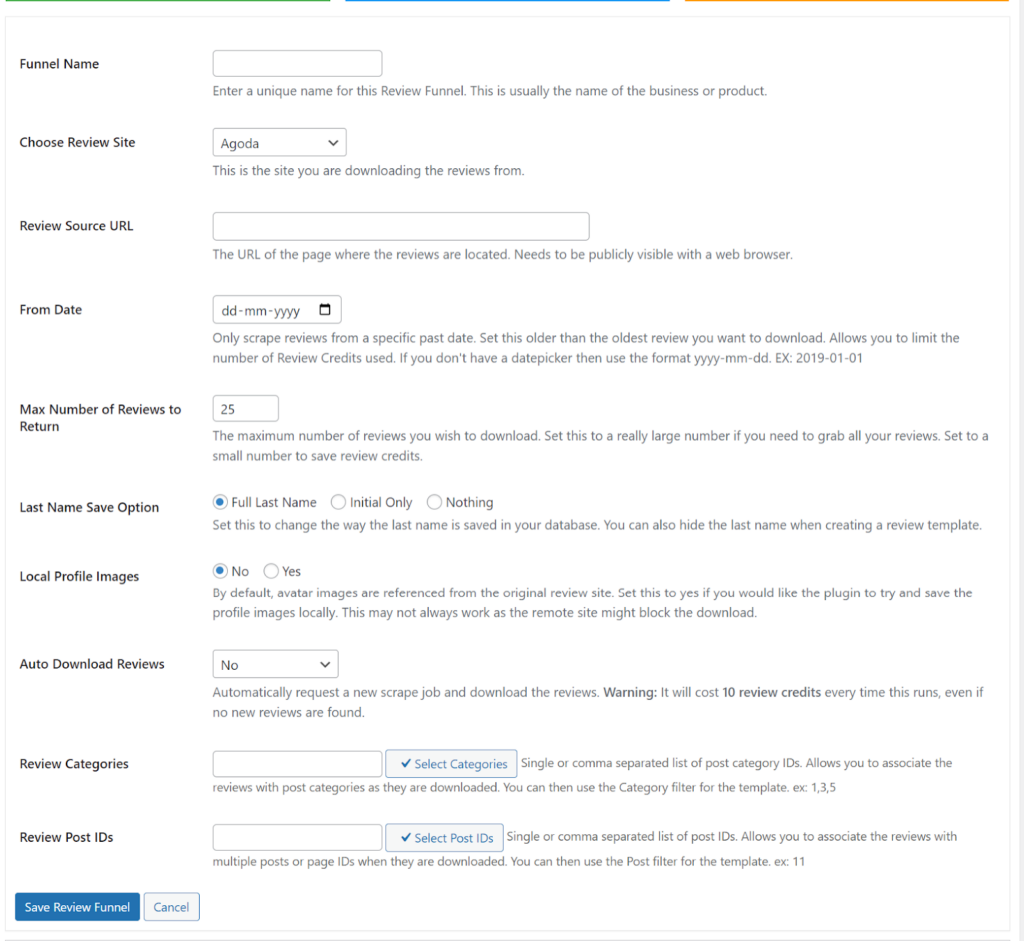**Detailed Caption for the Screenshot Image:**

The screenshot displays the top section of a web page related to setting up a review funnel. At the top, there are three colored progress lines: green on the left, blue in the middle, and orange on the right. The page is set up to configure the review funnel details. The first input field, labeled "Funnel Name," is currently empty, with a prompt stating, "Enter a unique name for the review funnel," typically the name of a business or product.

Below it is a section titled "Choose Review Site," where Agoda has been pre-selected from a drop-down menu, indicating that other review site options are available. A note explains that this is the site from which reviews will be downloaded.

Next, there's a field for "Review Source URL," which is also empty. Instructions specify that the URL should be publicly visible in a web browser. Another input, "From Date," allows users to scrape reviews from a specified past date, using the format year-month-date if there's no date picker available.

The field for "Max Number of Reviews to Return" is set to 25, with an explanation that this limits the number of reviews to download, allowing users to save review credits by setting a smaller number or grabbing all reviews by setting a large number.

Under "Last Name Display Options," the choice "Full Last Name" is selected from options that include "Initial Only" and "Nothing." This determines how last names are saved in the database and whether they are hidden when creating a review template.

Another toggle, "Local Profile Images," is set to "No," implying that avatar images will be referenced from the original review sites by default.

The "Auto Download Reviews" option is also set to "No," meaning that new scrape jobs will not be automatically requested and downloaded.

Lastly, there's a section for "Review Categories and Review Post IDs." At the bottom of the page, two buttons are displayed: "Save Review Funnel" and "Cancel."